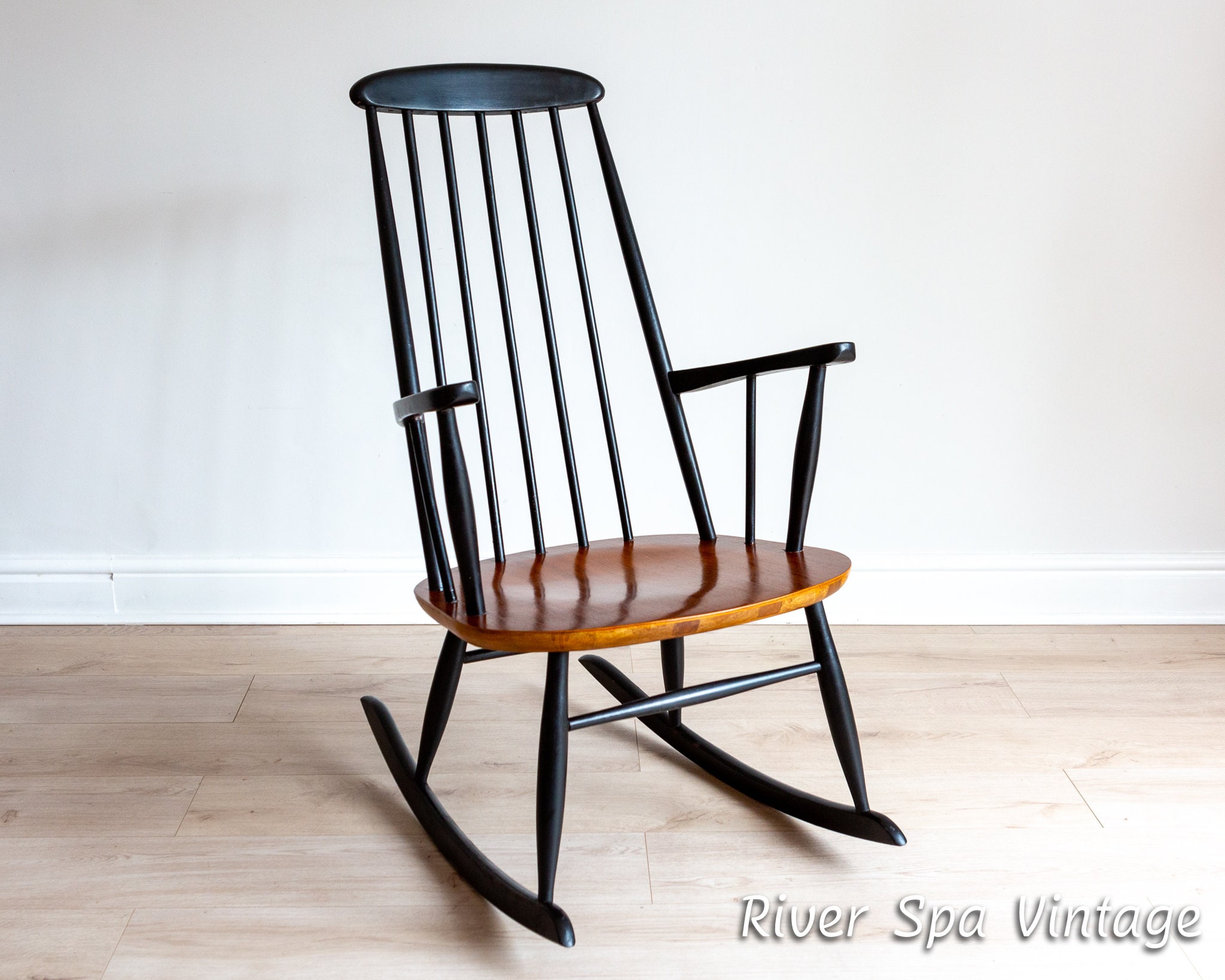The image depicts a wooden rocking chair positioned in the center of a room with white walls and light wood-colored flooring, likely laminate. The chair features a dark reddish-brown wooden seat, while the rest of the chair, including its two armrests and numerous horizontal and vertical bars forming the back, is painted black. The chair’s base consists of two curved wooden pieces enabling it to rock. The photo includes subtle text in the bottom right-hand corner stating "River Spa Vintage" in white font with black shadowing. The rocking chair is slightly angled towards the viewer, making its elegant and vintage design the focal point of the otherwise minimalistic room.